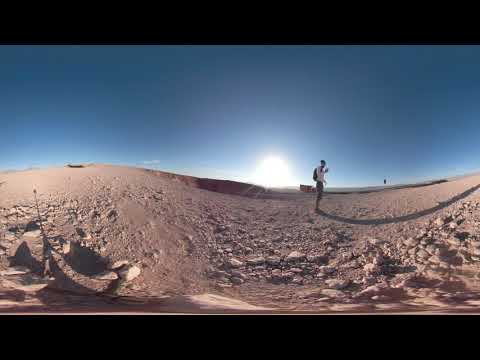In this image, a solitary figure stands in the distance of an expansive, barren desert landscape. The terrain features light brown and tan sand interspersed with grayish and white rocks. The person, clad in shorts, a white shirt or sweatshirt, and a backpack, faces away from the camera, holding an unidentified object in their hands. The scene is bathed in bright sunlight, with the sun positioned just right of center on the horizon, casting long and wavy shadows. The sky above is a clear blue with minimal clouds. Distant mountains and a possible low-lying structure or drone add depth to the deserted environment. The photograph appears slightly distorted, reminiscent of a 360-degree or fisheye lens, emphasized by the curving lines and wavy shadows. Horizontal black bars frame the top and bottom of the image, completing the letterboxed effect.